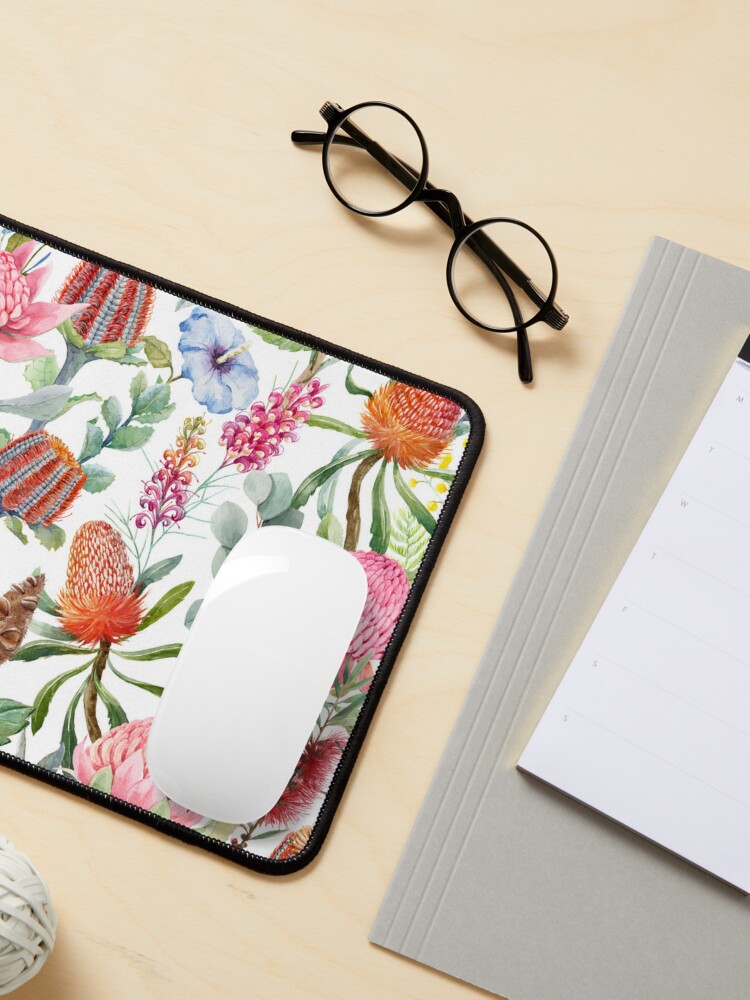This is a detailed top-down image of a light tan desktop scene. In the lower left corner, there is a white rubber band ball. Moving upward, there's a vibrant mouse pad adorned with a variety of colorful flowers on a white background, hosting a sleek, thin white Apple mouse. Above the mouse pad, a pair of thin, round black wireframe glasses are placed. To the right of these items, there's a thin gray notebook, topped with a notepad that has the initials of the days of the week and lines to organize a weekly schedule.